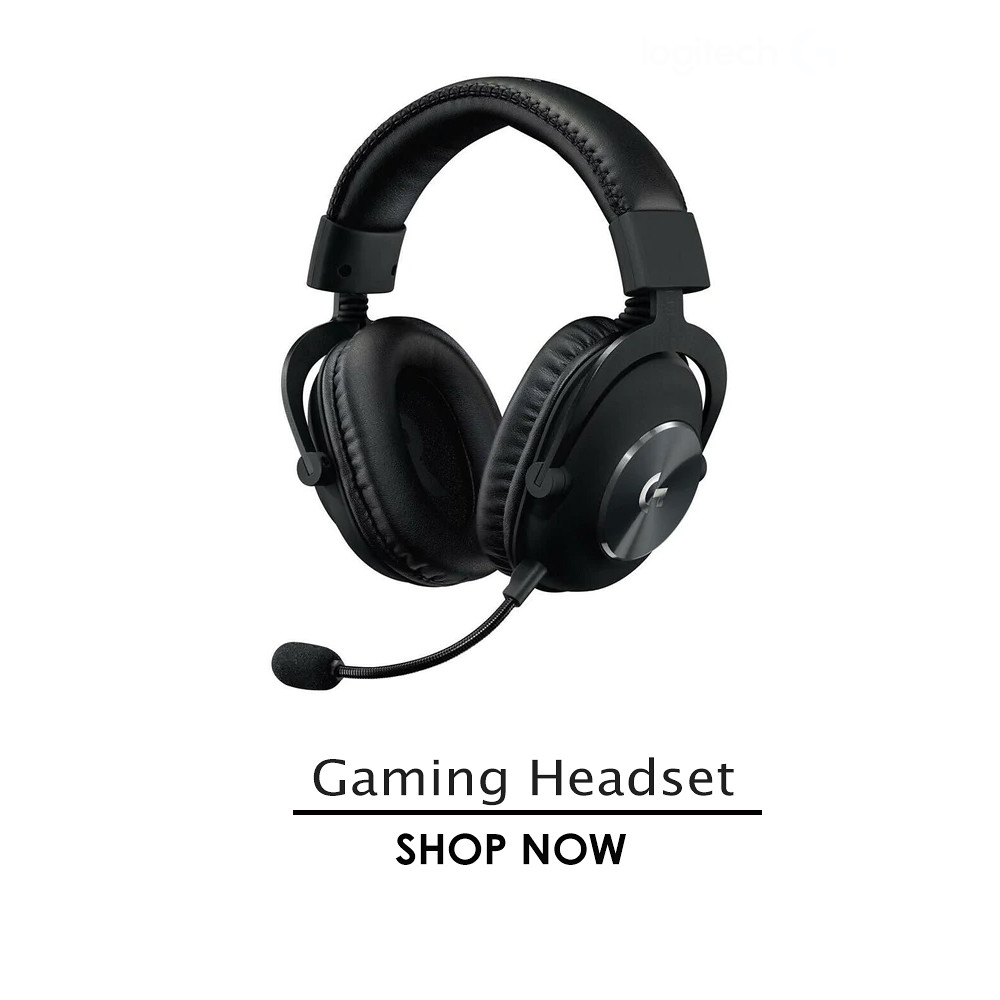The image displays a pair of black gaming headphones, set against a stark white background. These over-the-ear headphones feature a cushioned headrest and large, thick foam cups designed to provide comfort during extended use. Protruding from the left ear cup is a flexible, adjustable microphone. Each ear cup bears a notable G logo, which seems to belong to the brand. Directly beneath the headphones, the text "gaming headset" appears in regular lowercase, except for the capitalized "G" and "H," and a bold, uppercase "shop now" prompt. The overall design and the contrast against the white background make the details of these wireless, possibly leather or pleather, headphones particularly prominent.